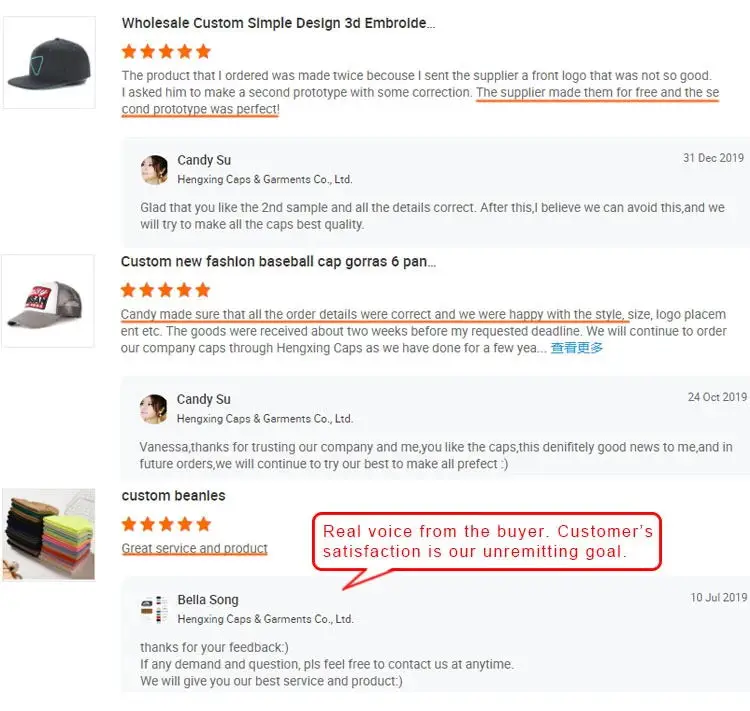Here is a cleaned-up and detailed caption:

---

**Image Description:**

The image depicts a section of a shopping website featuring three products: Custom Wholesale Simple Design 3D Embroidered Baseball Caps. Each product has received a five-star review from buyers. 

The first product, a custom baseball cap, is accompanied by a detailed customer review. The reviewer explains that they initially sent a less-than-ideal front logo to the supplier, which resulted in the product being made twice. Upon requesting corrections, the supplier remade the cap for free, and the second prototype was perfected. The supplier responded positively, expressing their gladness that the customer liked the revised sample and ensuring that future products would be of the best quality.

The second product, another custom baseball cap, has a review praising the attention to detail by a person named Candy and also features a five-star rating. The supplier responded with a generic thank-you message.

The third product, Custom Beanies, also holds a five-star review commending the great service and product quality. The supplier acknowledged the feedback with a thank-you note.

Additionally, there is a small talking bubble edited into the image, which states, "Real voice from the buyer: customer satisfaction is our unremitting goal," emphasizing the commitment to meeting customer expectations.